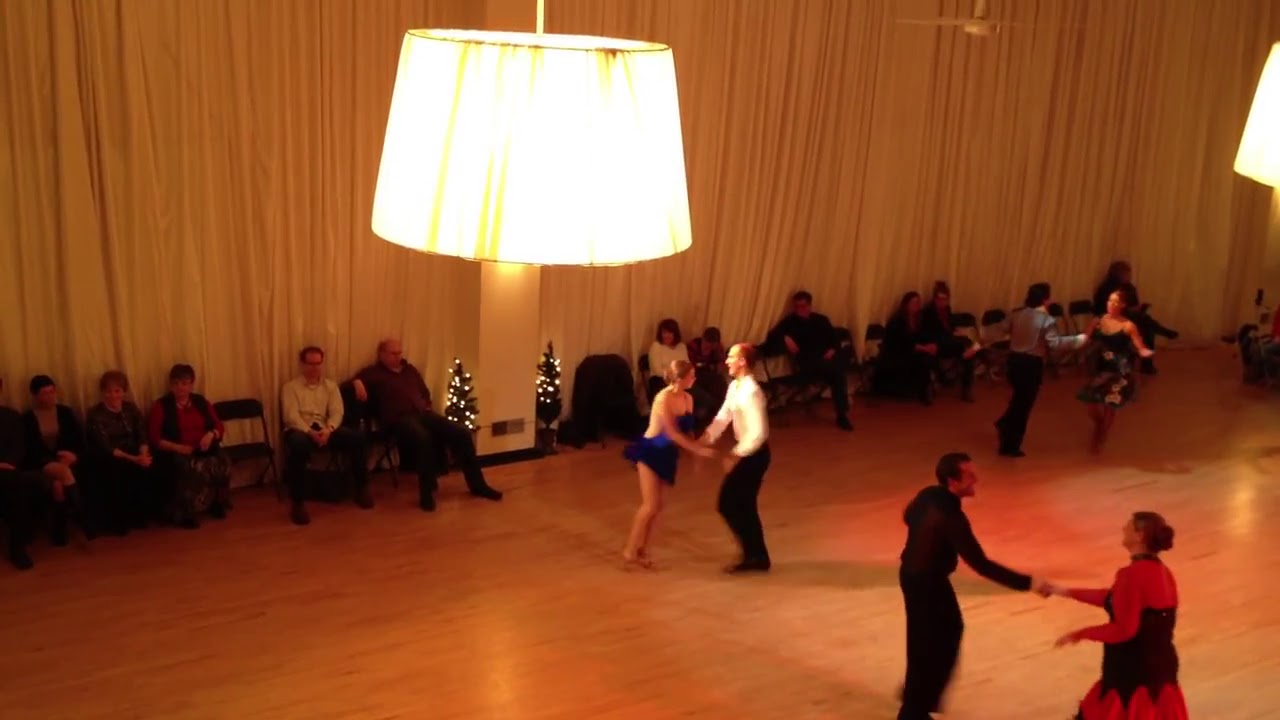The image captures an aerial view of a vibrant ballroom dance event set on a spacious hardwood floor. Couples, elegantly dressed in formal attire, are seen gracefully moving to the rhythms of what appears to be salsa or another type of sophisticated dance. Prominently, a man in a white shirt and black slacks partners with a woman in a dark blue dress, while nearby, a man in a black long-sleeve shirt dances with a woman in a red and black dress. Another couple features a man in a blue shirt with black slacks alongside a woman in a black dress adorned with white patchwork. The room is warmly lit by overhead lamps, casting soft shadows across the dance floor, enhancing the festive ambiance. Tall, cream-colored curtains drape along the walls, in front of which numerous guests are seated on folding chairs, attentively watching the dancers. Adding to the festive atmosphere, two small Christmas trees, illuminated with clear lights, are visible in the scene. The entire setting exudes a celebratory vibe, with everyone appearing to revel in the joyous occasion.